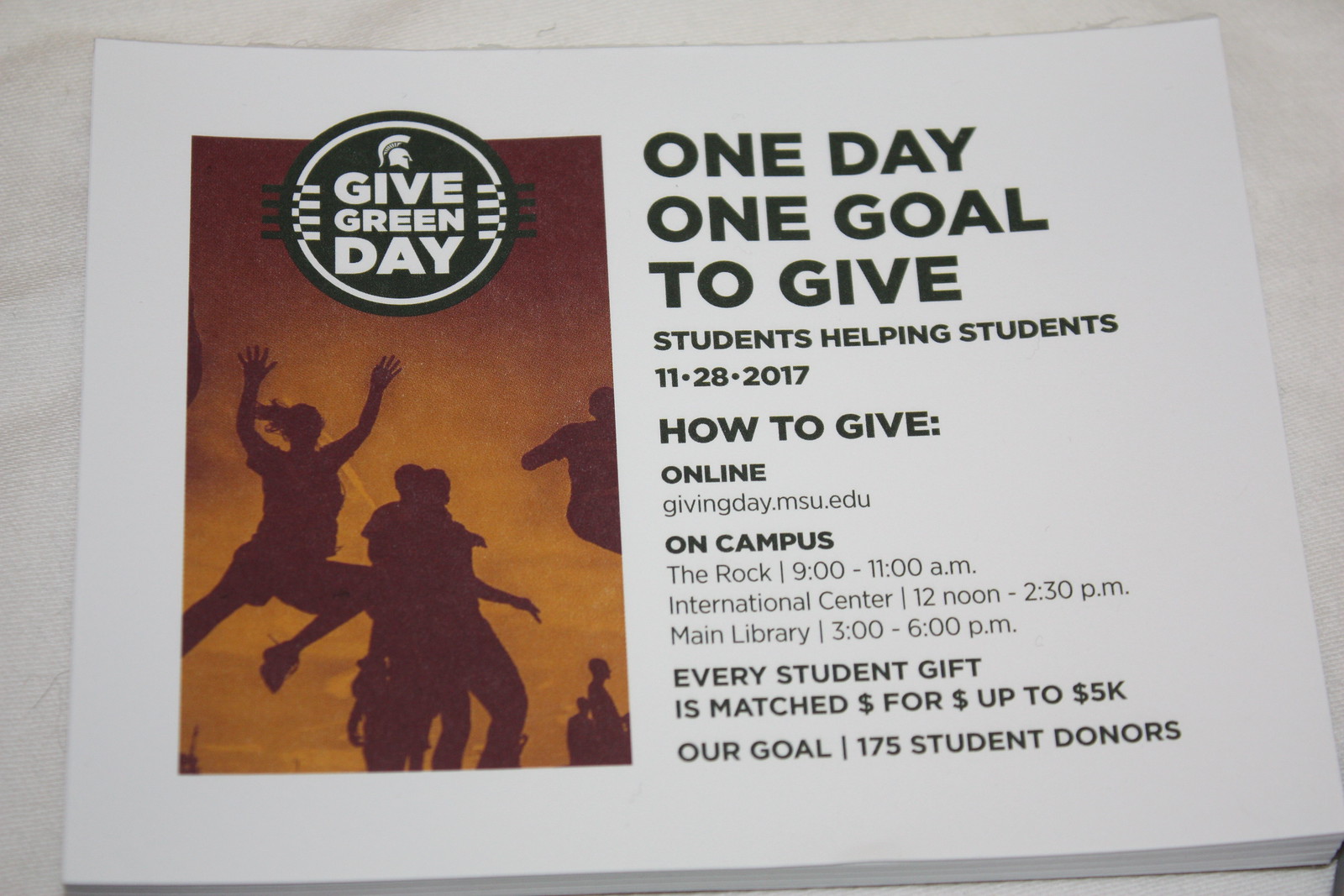This image features a detailed flyer advertising a college event called "Give Green Day". The flyer appears to be set against a plain white background, with the entire scene captured in a landscape orientation. 

On the left side of the flyer, there is a vertical rectangle with a light brownish-orange background showcasing the silhouettes of people in dynamic poses, including one person jumping from left to right. Above these figures, a green circle containing a white Trojan helmet logo is depicted, signifying the event's branding. 

To the right of this visual element, bold black text on a white background declares the event details: "One Day, One Goal, To Give - Students Helping Students." The flyer specifies the date as November 28, 2017, and outlines how supporters can contribute: online at givingday.msu.edu or in-person at several campus locations including The Rock from 9:00 to 11:00 a.m., the International Center from noon to 2:30 p.m., and the Main Library from 3:00 to 6:00 p.m. It highlights that every student's donation will be matched dollar for dollar up to $5,000, with a goal of reaching 175 student donors. The flyer utilizes colors like off-white, red, yellow, orange, green, and black to attract attention and convey its message.